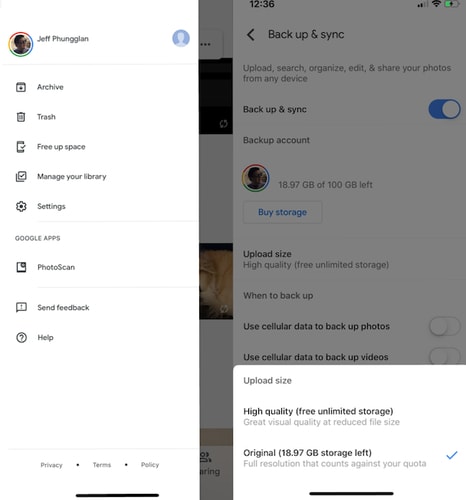The image depicts a detailed screenshot of Google settings, specifically tailored for the user Jeff Phungglan. The left-hand side features a sidebar menu with the user's profile picture, encased in a border reflecting Google's signature color scheme. Below the profile picture, there are several icons and links, including options such as "Archive", "Trash", "Free up space", and "Manage your library settings".

Further down the sidebar, there's a section labeled "Google Apps", which lists "PhotoScan" as the only available app. Additional utility links like "Send feedback" and "Help" are also present. At the very bottom, options concerning privacy, terms, and policy are found.

The primary section of the screen captures another settings page, designated for "Backup and Sync". This section is somewhat grayed out, indicating it might not be the focal point of current activity. Overlaying this screen is a prominent white pop-up window detailing "Upload size" options. The options include:

1. **High quality** (Free unlimited storage) - Offers great visual quality at a reduced file size.
2. **Original** (18.97 GB storage left) - Provides full resolution uploads that count against the user's storage quota.

The "Original" option is selected, marked by a distinct blue checkmark. The overall layout and content suggest this is a settings page centered around managing photo and video backups and synchronization with Google services.